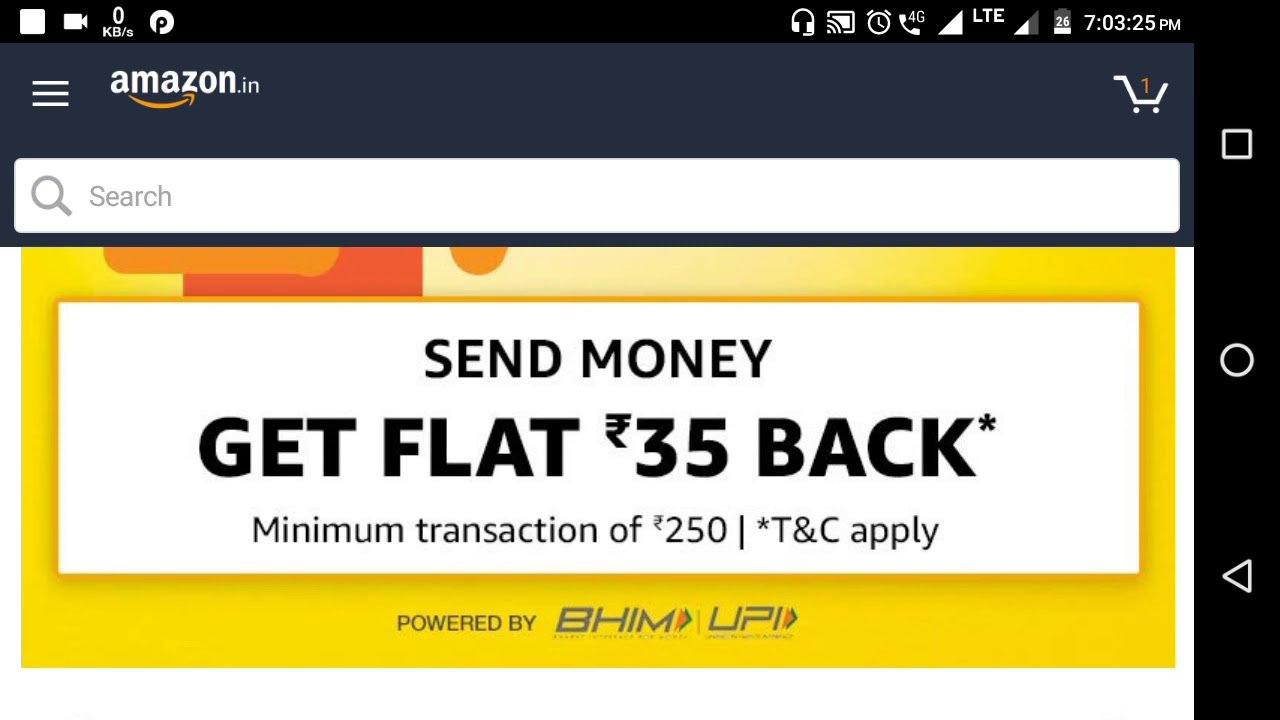The image captures a smartphone held in landscape orientation, evident by the phone's option keys visible on the right side. The screen displays the Amazon website, as indicated by the Amazon logo in the top left corner. Directly below the logo is a blank search bar. In the top right corner, an icon of a shopping cart is shown with a notification indicating one item inside.

Prominently displayed on the screen is a promotional banner with a yellow background, advertising a cashback offer: "Send money, get flat $35 back, minimum transaction of $250. Terms and conditions apply." At the very bottom, it notes that the service is "powered by BHIM UPI."

At the top of the screen, the time is shown as 7:03:25 PM. Additional status icons provide information including signal strength, LTE network connection, 4G capability, and the battery level, which is at 26%.